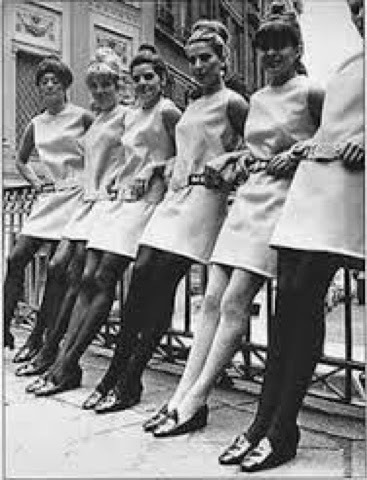This black and white photograph depicts six women leaning against a railing at what appears to be a water fountain. All of the women are dressed in matching white, sleeveless, high-neck dresses that hit around mid-thigh. They present a poised and serious demeanor, perhaps indicative of the formal context or their purposeful roles. Their hairstyles, which are evocative of the 1960s, are all up in buns except for one woman on the far left whose hair is styled differently. Notably, their footwear consists of shiny black loafers with a slight heel, adding a touch of elegance. They appear fashionable and determined, further emphasized by their immaculate shoes. The four women on the left side of the photograph wear dark-colored tights, while the two on the right do not. Behind them, portions of buildings can be seen, creating a subtle urban backdrop. The overall scene evokes a sense of vintage sophistication and composure.